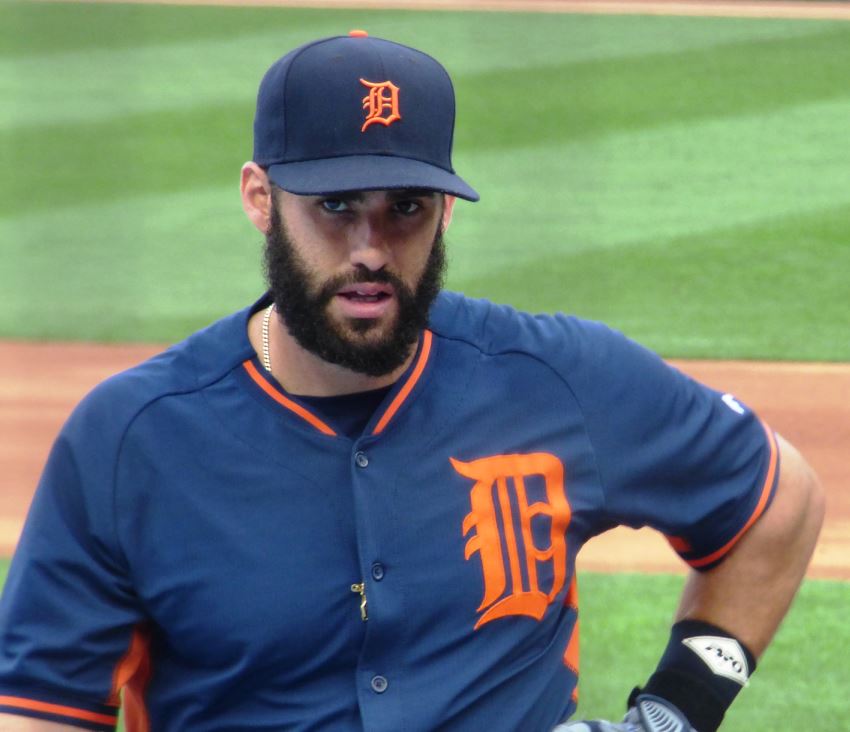The image features a handsome baseball player with a thick black beard and mustache, possibly biracial but described by some as white. He stands looking slightly beyond the camera with a confident expression. He wears a navy blue baseball cap with an orange 'D' in old-style English font at the center. His navy blue jersey, adorned with an orange 'D' on the left chest, features orange trim around the collar and short sleeves ending above the elbow. He also sports a black and white wristband on his left wrist and a gray glove. The background reveals the green grass of the outfield and the brown dirt of the baseball diamond, suggesting the setting is a baseball field.